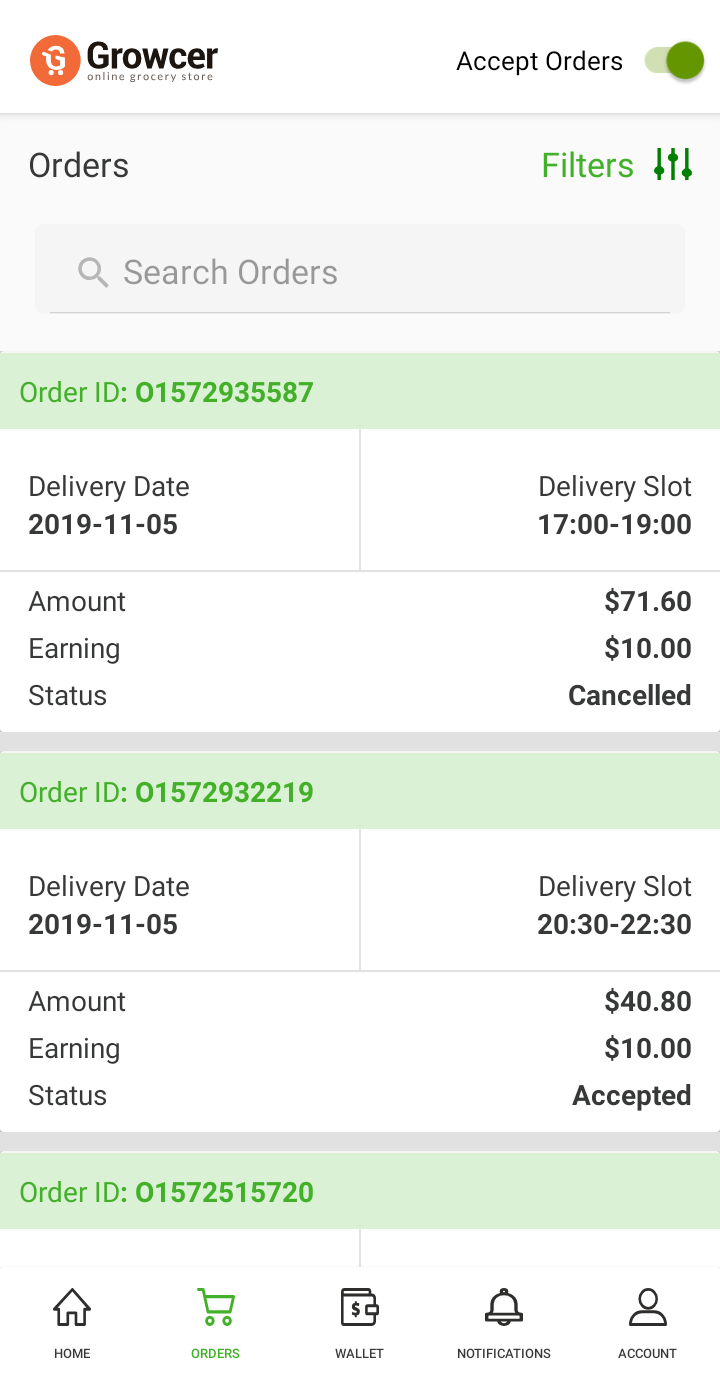The image depicts a screenshot of the homepage of Growcer, an online grocery store platform. In the top left corner, the logo "Grocer," spelled "G-R-O-W-C-E-R," is prominently displayed, accompanied by a tagline underneath that reads "An online grocery store." The icon for Growcer is an orange circle featuring a stylized letter "G" merged with a shopping cart graphic. 

Next to the logo, there is an option labeled "Accept Orders" with a toggle switch to enable or disable this feature. Below this top section, there are several distinct boxes and controls. 

The first box is labeled "Orders" and adjacent to it is a "Filters" option, which includes a drop-down menu for refining the search. Further below, there are options and a search bar labeled "Search Orders."

The next box has a green background and includes detailed information about an order. It lists the order ID: "0157-2935587," the delivery date, delivery status, and slot time and date. Additional details include the amount and earning status for the order.

The subsequent box contains similar information for another order: it displays the order ID, delivery date, delivery slot, amount earning status.

The final box provided includes another order ID number but lacks details such as the delivery date and slot, along with other specifics.

At the bottom of the page, there is a menu bar featuring icons with corresponding labels: 
- Home with a house icon
- Orders with a shopping cart icon
- Wallet with a wallet icon
- Notifications with a bell icon
- Account with a stick figure icon